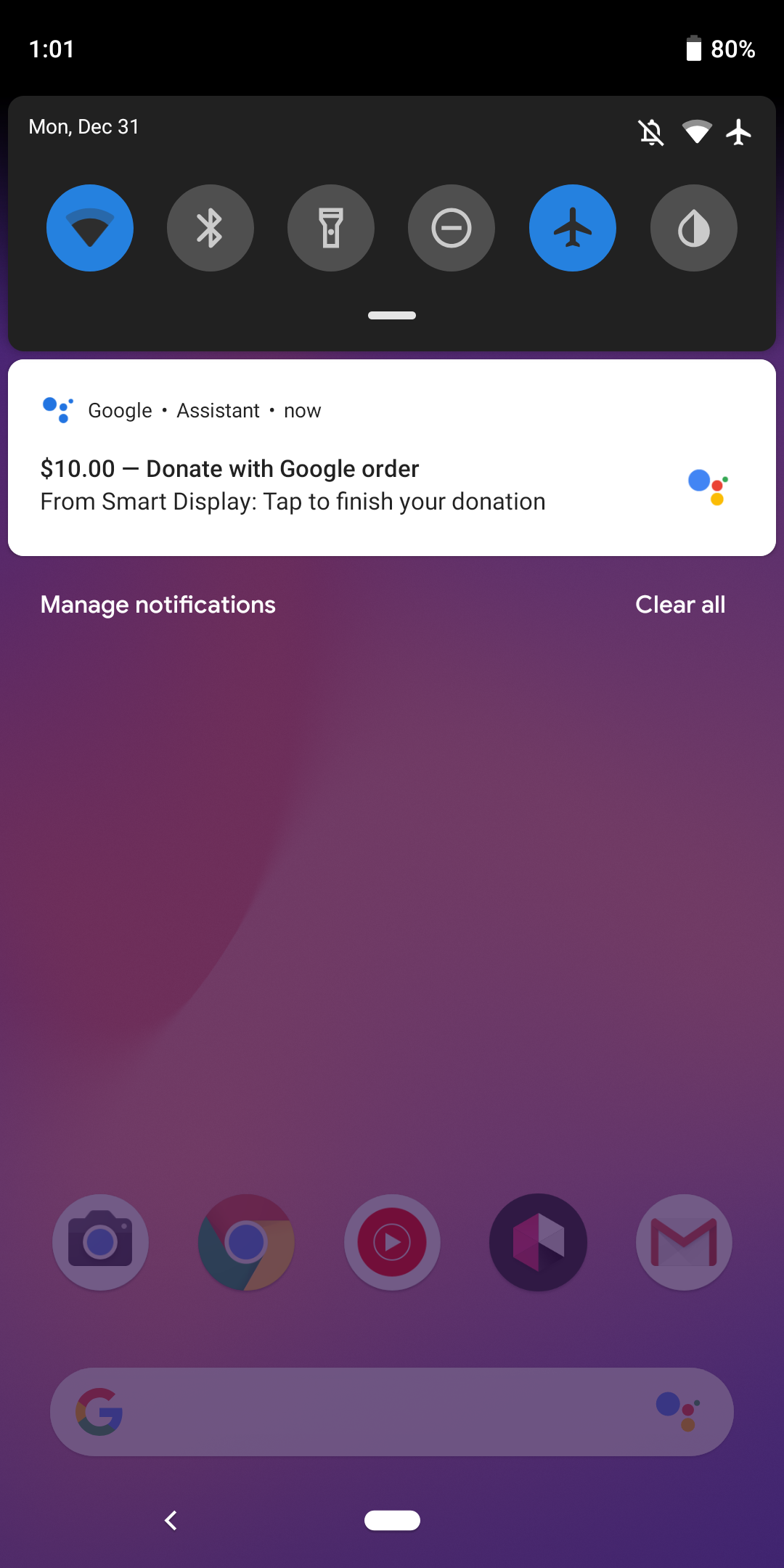This screenshot, captured in portrait mode from a cell phone, presents a detailed view of the device's user interface on Monday, December 31st. 

At the top, against a black background, the status bar displays essential icons: the time "10:11," a Wi-Fi signal, and a battery icon indicating 80% charge. Below this, a lighter black banner prominently shows the date "Monday, December 31st" on the left, and notification indicators on the right, stating "No notifications" and "Airplane mode."

The next row features six circular icons, where the Wi-Fi and Airplane Mode icons are highlighted in blue. Following these icons, there's a notification from Google Assistant stating: "Google Assistant: Now $10 donate with Google. Order from Smart Display. Tap to finish your donation."

The background transitions to an abstract blend of purples with various shapes. Directly under the notification, options to "Manage notifications" on the left and "Clear all" on the right are visible.

At the very bottom of the screenshot, several app icons are lined up, including the Camera, Google, an app with a red circle, another unidentified black app, and Gmail. Below these icons, a Google search bar appears, signifying that the user may be preparing to search or manage their apps and settings on their phone.